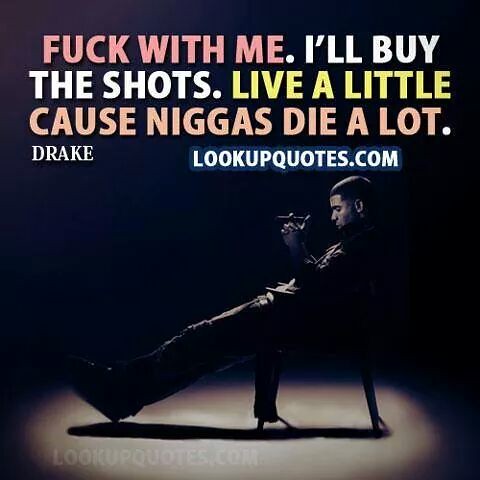The image resembles a Drake meme or possibly an album cover featuring the musician Drake. The background is black, and a spotlight illuminates the central figure, Drake, who is seated on a chair. Drake, clad in a dark long-sleeve top, dark trousers, and black shoes, is holding a cigar in his right hand. His head is angled downward, suggesting a contemplative pose, with his legs stretched out and crossed at the ankles. Above him, a quote reads, "F with me, I'll buy the shots. Live a little, 'cause people die a lot." The text is displayed in varying colors—pink, yellow, and white. Below the quote, the text "lookupquotes.com" is also visible. The spotlight casts a dramatic effect, silhouetting Drake against the dark background, making him the only illuminated figure in the image.